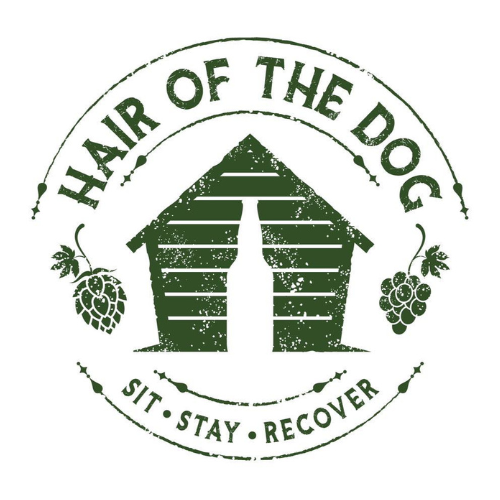This logo features a vintage, circular design rendered entirely in dark green. The logo's circular shape is formed by two separate, ornate semicircles on the top and bottom that do not meet at the sides, creating an open feel. Inside this outer circle, the top arc contains the text "Hair of the Dog" in curved letters, while the bottom arc reads "Sit, Stay, Recover." Both phrases are in capital letters and follow the circular contour.

At the heart of the design stands a doghouse, characterized by vertical slats. The entryway of the doghouse is cleverly shaped like a beer bottle, emphasizing the logo's theme. To the left of the doghouse is an image of hops, complete with leaves, and to the right is a vine of grapes. The entire illustration has a slightly faded and worn texture, giving it a rustic, old-timey appearance. The background of the image is white, accentuating the green hues and making the elements of the logo stand out clearly. This could potentially be a logo for a tavern, brewery, or a product related to alcohol recovery.